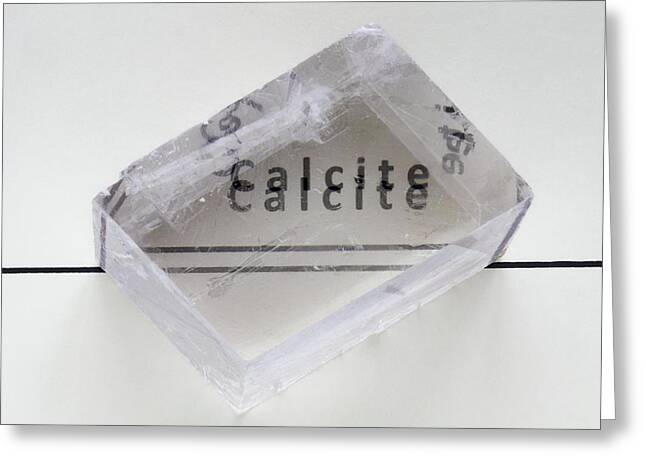This photograph showcases a piece of CalSight, a translucent carbonate mineral prominently featured in the image. The word "CalSight" is visible twice within the mineral, giving a mirrored effect. The CalSight itself is shaped like a brick with rounded corners, spanning from the lower right corner to the upper right corner against a baby blue-gray background. The mineral, which appears almost folded like a card, has two thin horizontal lines running through its center, transitioning into a single black line at the edges. The various shades of gray and white on the object, along with the reflection of the lettering on its side walls, create an intriguing visual layered with depth and texture.